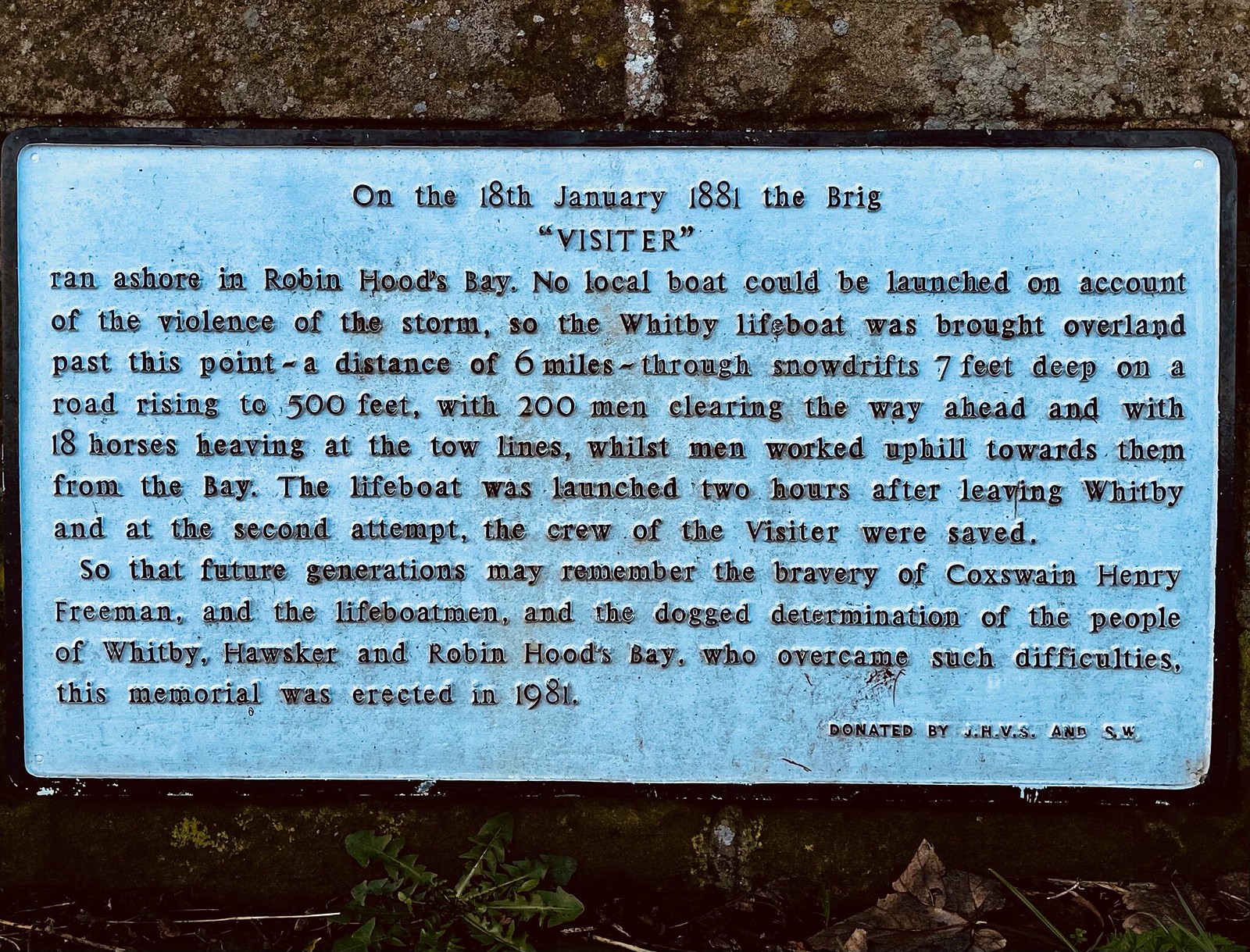The image depicts a memorial plaque mounted on a stone background. The plaque itself is light blue with a black outline and black text. It commemorates a remarkable rescue event that took place on January 18, 1881, when the brig "Visitor" ran ashore in Robin Hood's Bay during a violent storm. Due to the intensity of the storm, local boats were unable to launch, prompting the Whitby lifeboat to be transported overland for six miles through snowdrifts seven feet deep, on a road inclining to 500 feet. This formidable journey involved 200 men clearing the path and 18 horses towing the lifeboat, while men from the bay worked towards them uphill. The lifeboat was successfully launched two hours after departing Whitby, and on its second attempt, the crew of the "Visitor" was rescued. This plaque honors the bravery of Coxman Henry Freeman, the lifeboatmen, and the unwavering determination of the people of Whitby, Hawker, and Robin Hood’s Bay. The memorial was erected in 1981, donated by J.H.V.S. and S.W. In the photograph, the sign is shown in a landscape orientation, mounted between two large tree trunks that are partially visible at the top and bottom edges, enhancing the detailed realism of the scene.